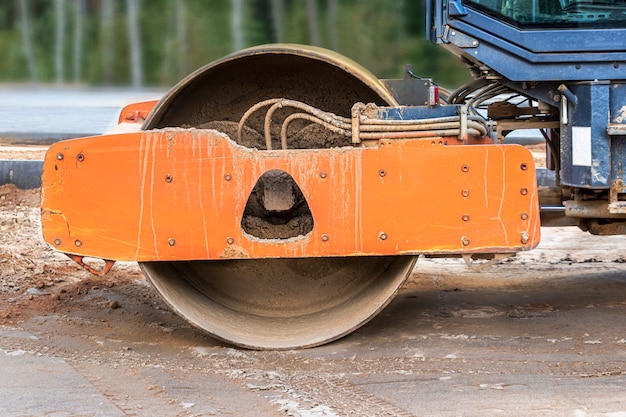This is a detailed color photograph capturing the back section of a road roller, traditionally known as a steamroller, used for flattening pavement. The focus is on the metal wheel of the roller, which is cylindrical, hollow, and viewed from the side. An orange metal plate, adorned with multiple rivets, is positioned in front of the wheel, serving as a distinct barrier. Just ahead of the wheel, part of the cab of the machine is visible, showcasing a blue metal body with a window in the upper right corner, suggesting it has a glass compartment for the driver. The ground beneath the roller appears to be a paved surface with some dirt, adding texture to the scene. In the background, an asphalt layer stretches across, partially bordered by a forest with white birch trees and lush green foliage, all under a cloudy sky that casts no shadows.